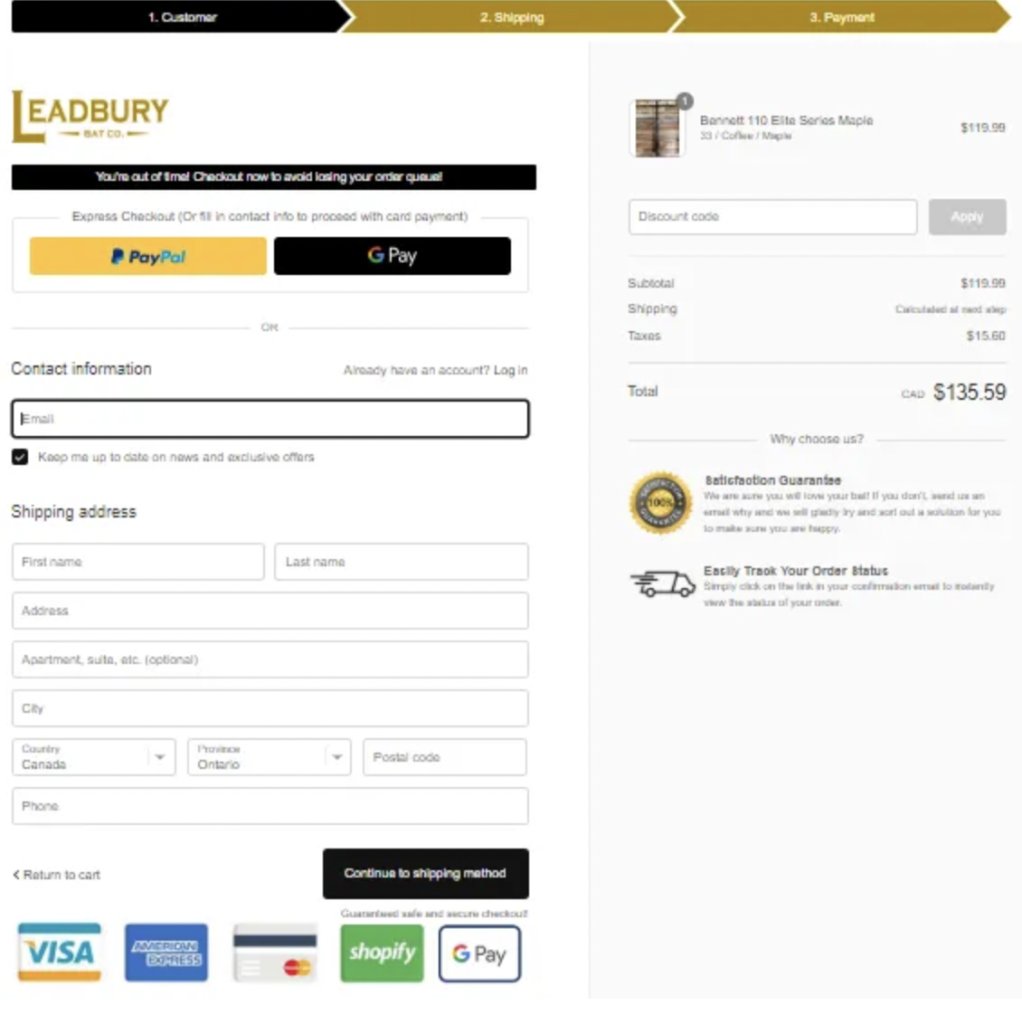Image Caption:

"Screenshot of an online checkout page displaying the process to complete a purchase. The page involves multiple steps including filling in contact information and selecting a payment method. Users have the option to pay via card (Visa, American Express, Discover), PayPal, or Google Pay. The form requires details such as first name, last name, address (including premises and suite, if applicable), city, country (Canada), province (Ontario), postal code, and phone number.

The checkout card reflects a summary of items being purchased, specifically showing 'Benet 110 Elite Series Maple' priced at $119.99 CAD. A black rectangle button labeled 'Continue to Shipping Method' is prominently displayed for proceeding to the next step. Below the item summary, the subtotal is listed as $119.99 CAD, with an additional shipping charge and taxes amounting to $15.60, bringing the total to $135.59 CAD.

There is an emphasis on Express Checkout options provided at the top right corner of the page, and a section for inputting a discount code. Additionally, a notification emphasizes easy order tracking capabilities. Overall, the interface aims to ensure a streamlined and secure payment experience for the user."